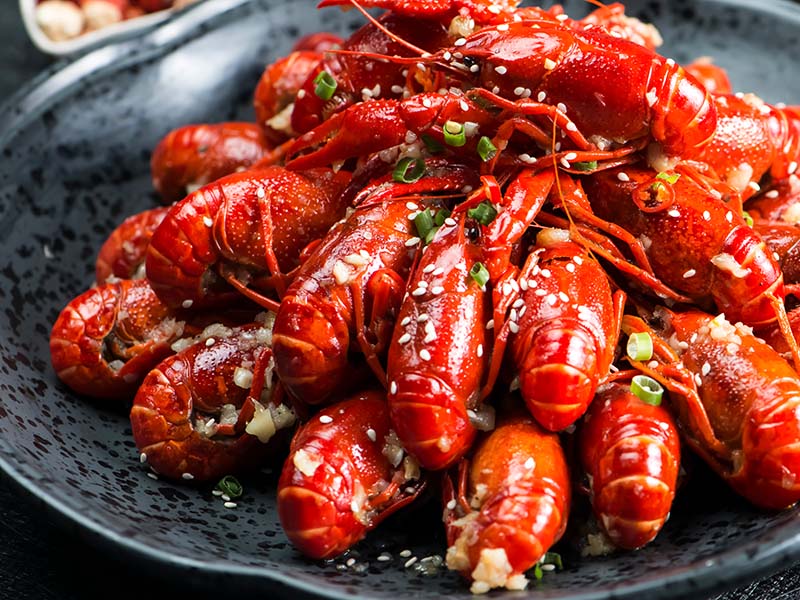In this close-up, color photograph, a vibrant pile of red crawfish is displayed on a shiny, gray metal platter with a black speckled pattern. Each crawfish is visibly detailed, showcasing their curled-up tails, spiny legs, and antennas, indicating they have been cooked. The dish is attractively garnished with scattered sesame seeds, chopped green asparagus, and pieces of garlic cloves, enhancing the visual appeal. The crawfish are very shiny, emphasizing their freshness and preparation. In the background, a secondary white dish containing more food is partially visible, suggesting a larger feast in progress.